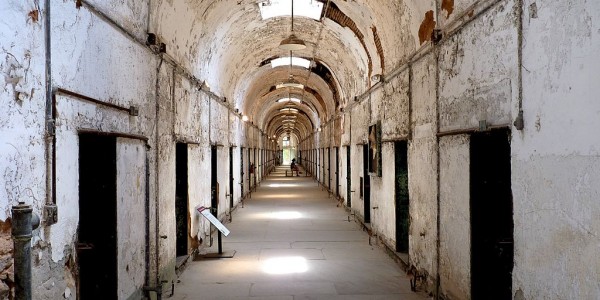The image depicts a lengthy, arched corridor that appears to be inside an old, abandoned building, possibly a prison. The sidewalls are a weathered white concrete, showing significant distress and decay. The ceiling is rounded and features a series of skylights that illuminate the hallway. The floor is covered with gray tiles, enhancing the corridor’s cold and eerie atmosphere. Along the right side of the corridor, as well as the left, there are dark, possibly metal doors without windows. The area above the doorways is cluttered with exposed pipes and wiring, all converging into a higher cable running the hallway's length. The corridor seemingly stretches endlessly, emphasizing its desolate and forsaken state. Near the far end, there appears to be a person seated in a chair in the middle of the hallway. On the left wall, there is an information sign, white with a black stand, adding to the impression that this building may have once served a functional, institutional purpose.